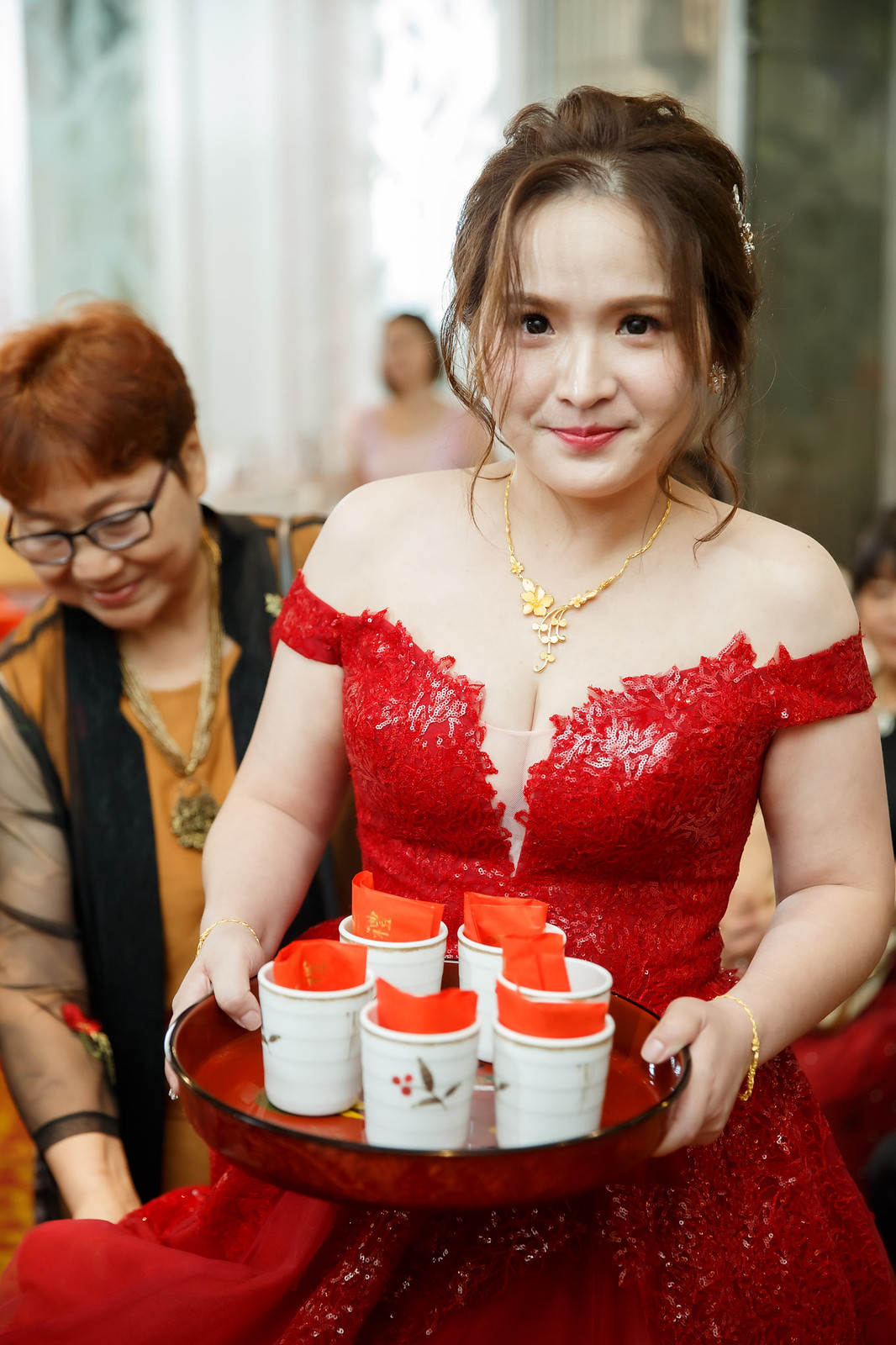This is a detailed color photograph of a young Asian woman with pale skin and brown hair styled in an elegant updo, with tendrils framing her face. She wears minimal yet tasteful makeup and lipstick, enhancing her delicate features. The woman is adorned with a gold necklace featuring a flower design pendant and a gold bracelet on her left wrist. Her attire is a stunning, red, lacy, off-the-shoulder gown with short sleeves, featuring red sequins and an illusion net panel for modesty between the breasts.

In her hands, she carries a round, red lacquer tray holding six small white cups, each with intricate designs of leaves and red berries, and containing folded red napkins or pieces of paper. The elegant and ceremonial nature of her ensemble suggests that she is preparing for a formal event, possibly a celebration or a reception.

Behind her stands a woman with short, dyed reddish hair and black glasses, who appears to be assisting by adjusting the train of her gown. This older woman, likely her mother, looks happy, reflecting a joyful atmosphere. The scene is completed by sheer curtains over a brightly lit window in the background, hinting at a lively gathering with more women whose faces are seen in the blurred background. The overall setting suggests a well-decorated and festive venue.